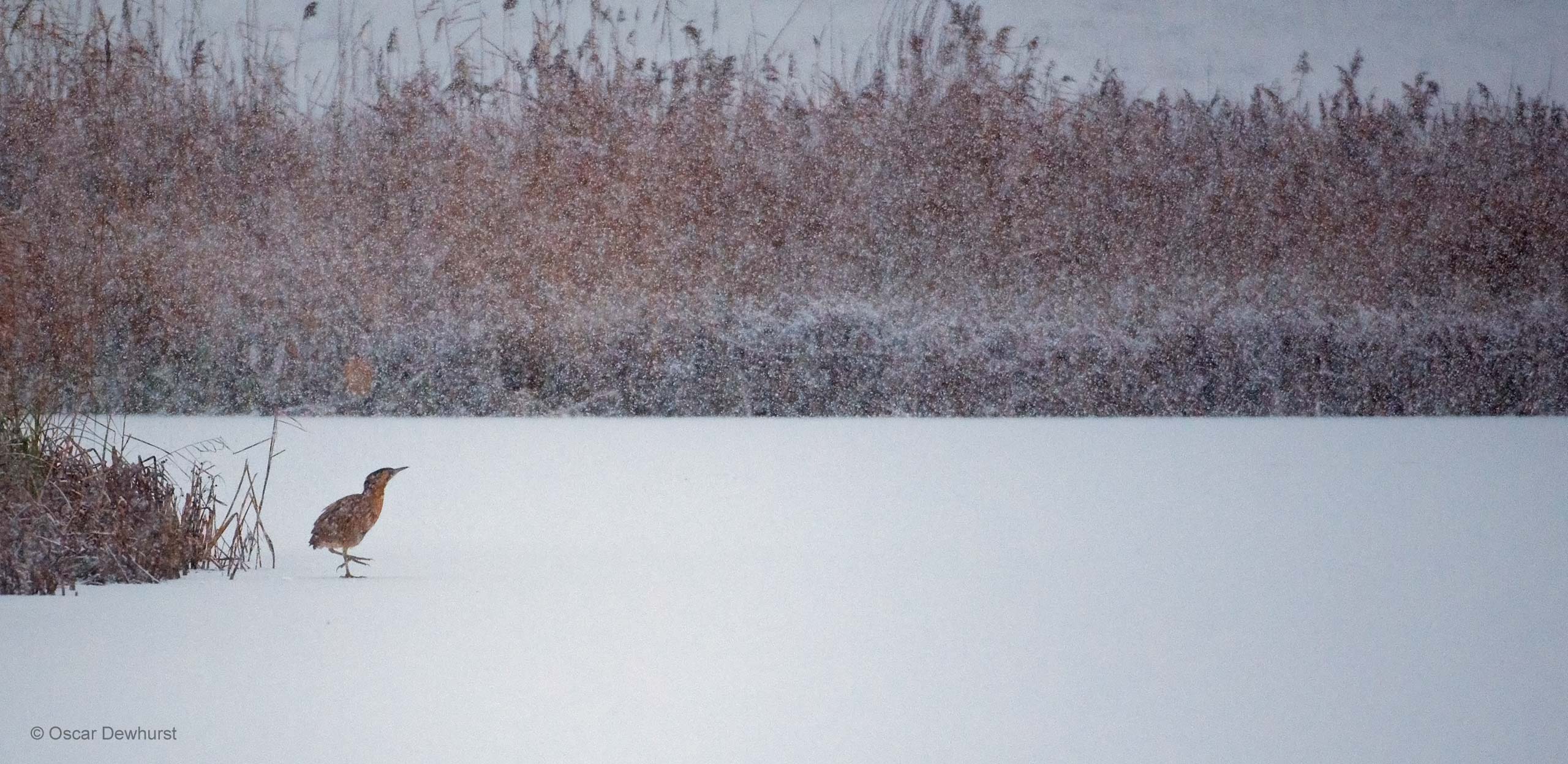This detailed photograph, captured outdoors in a horizontal landscape orientation, depicts a serene winter scene. The foreground features a flat, snow-covered surface that could possibly be a frozen pond. Stretching from left to right, this snowy expanse is pristine and untouched. 

On the lower left side, towards the bottom of the image, a small bird is poised mid-step on the snow. The bird, likely a sparrow, is facing to the right, with its right side visible. Its beak is pointed upward, suggesting alertness, and its left foot is lifted as if it's about to continue walking. The bird has a subtle yellowish hue, although it primarily appears brown.

Surrounding this snowy field is an array of brush and tall grasses, covered in a layer of snow. The brush, resembling cattails and reeds, provides a mix of golden wheat, rust, purple, green, and white colors. Some of these elements suggest that the snow may still be gently falling. 

In the background, the landscape is framed by a dense row of these tall grasses, adding texture and depth to the scene. The sky above is a uniform white, enhancing the wintry ambiance.

In the bottom left corner of the image, a watermark reads "Copyright Oscar Dewhurst," marking the photographer's work.